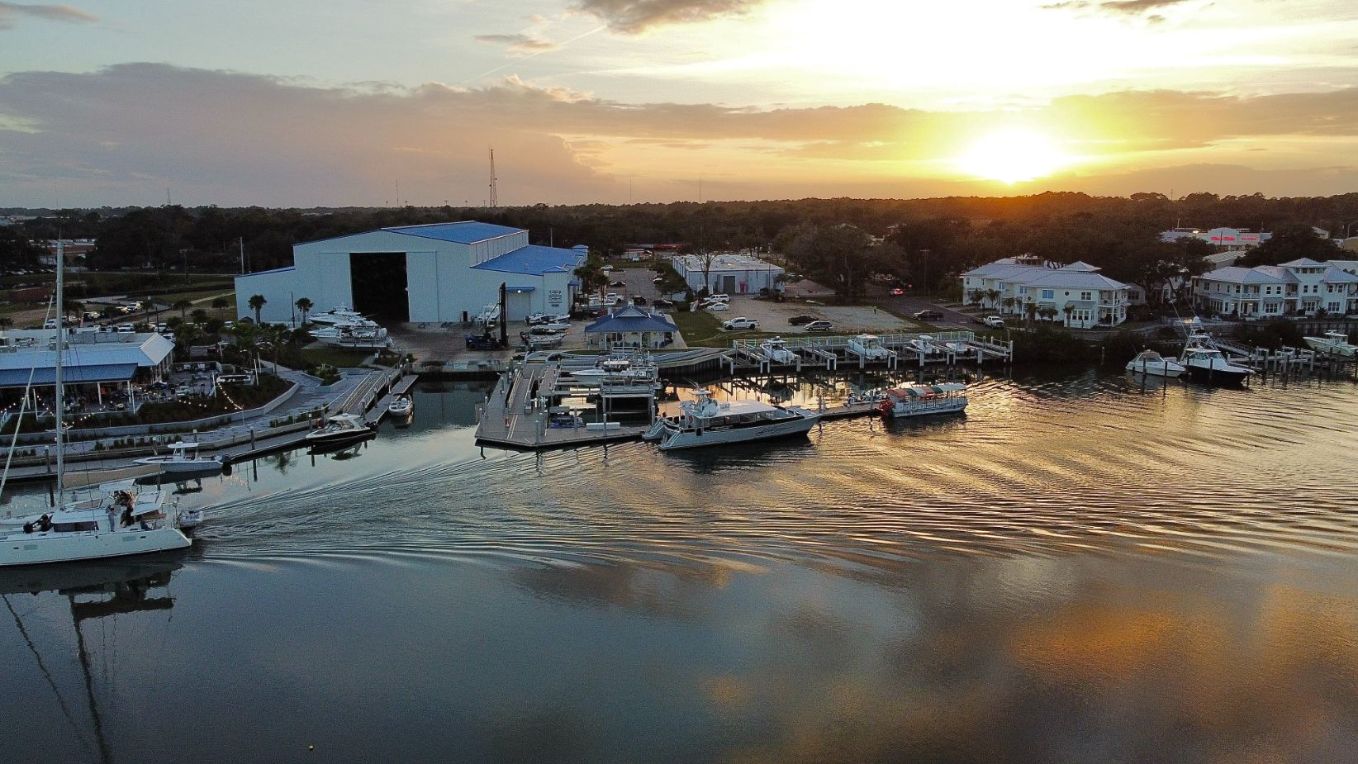This is a panoramic photograph capturing a serene marina at sunset in a small town. The calm water, with gentle ripples from a boat moving across, is dotted with an array of boats, most of which are white, including several yachts and smaller boats clustered around them. To the left, a large white warehouse with a blue roof stands prominently by the water's edge. On the right, further back, there are clusters of condos and large beach houses. The marina itself is defined by its docks and piers where boats are parked. Encircling the marina are drives or roads, and beyond it, a dense backdrop of trees reaches into the horizon. The sky above is painted with the vibrant hues of a sunset, with the sun just below the horizon, creating a striking contrast against the clouds.